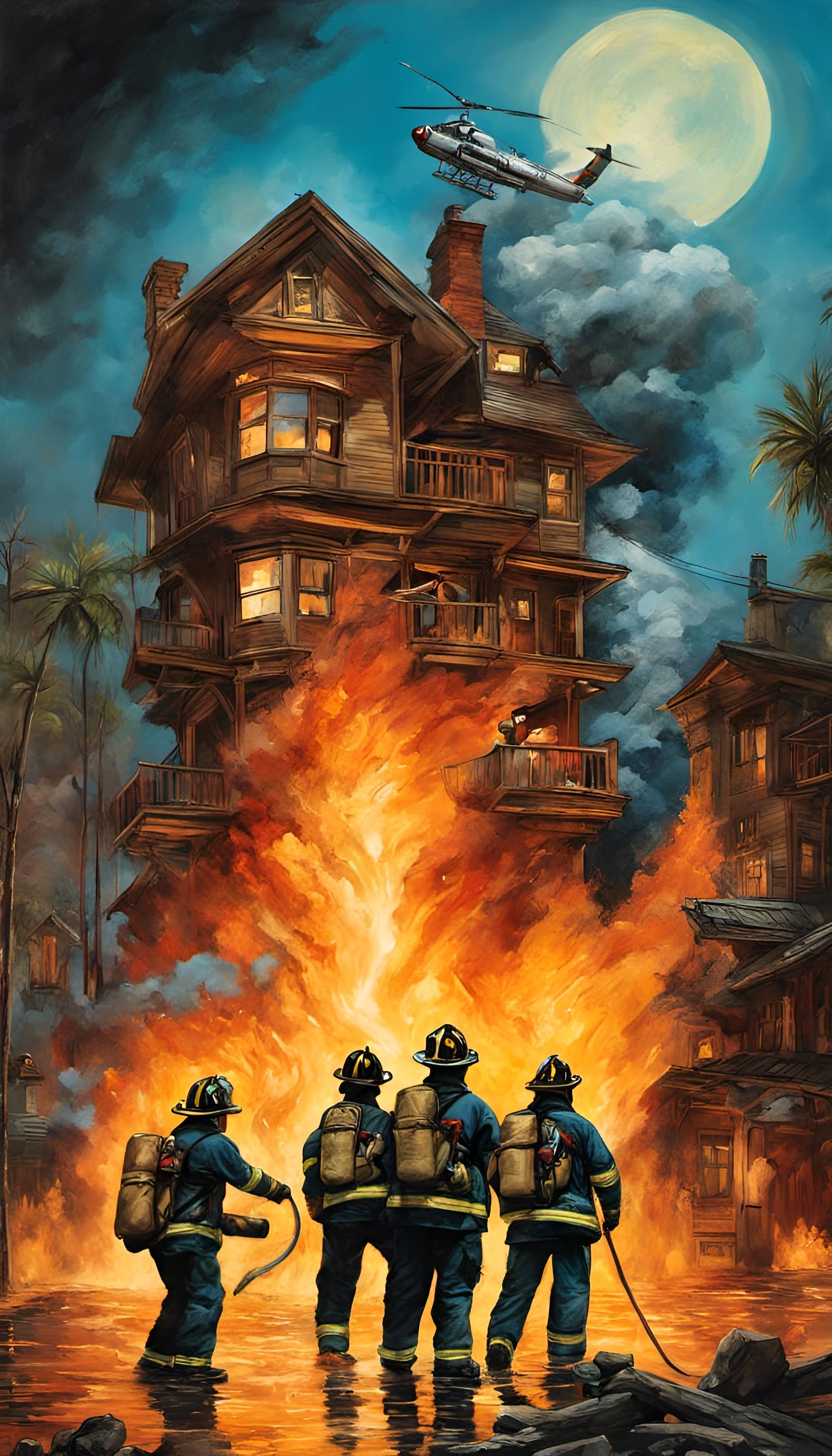The image depicts a vividly colored, likely AI-generated watercolor painting of an extraordinary six-story wooden house engulfed in flames. The scene is set at night, illuminated by a bright blue sky with a prominent moon situated at the top right corner. Amidst the billowing smoke, a helicopter hovers above, seemingly assisting in the firefighting efforts. The fire, which originated in the middle of the fantastically constructed house, is spreading rapidly to an adjacent building on the right, further intensifying the chaos.

In the foreground, four firefighters, outfitted in reflective gear and hats, stand in water, their figures mirrored in the fiery reflection below. Two of them appear to be holding hoses, though these seem disconnected due to the nature of the artwork. The house itself, with palm trees framing each side, is not only burning from the bottom up but also shows signs that there might be individuals on the balconies waiting to be rescued. The overall composition evokes a dramatic, almost fantasy-like portrayal of a night-time firefighting operation against a fantastical backdrop.